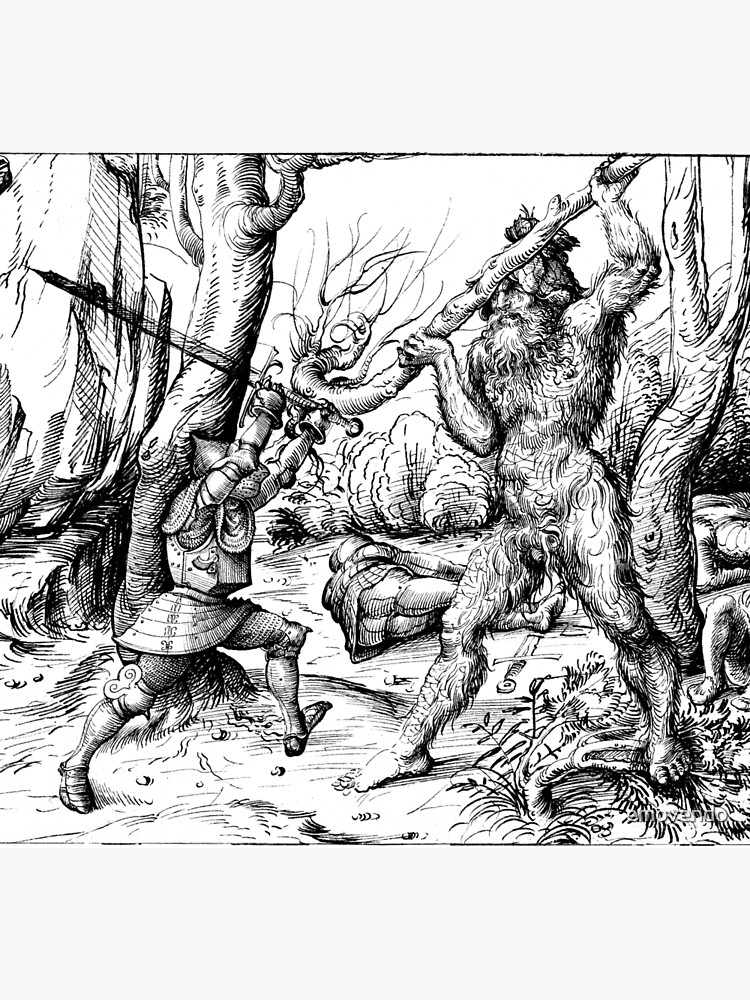This black and white drawing, rendered in ink, depicts an intense combat scene set within a forested area. The square illustration showcases a knight, fully armored from head to toe in chain mail and plate armor, positioned on the left. He brandishes a sword with both hands, poised to attack. Facing him on the right is a towering, monstrous figure resembling a yeti. This giant, nude, and incredibly hairy creature clutches a hefty wooden log raised above its head, as if about to bring it down on the knight. The creature's form is detailed with pronounced fur, and a small, barely noticeable penis can be seen. On the ground behind the combatants lies a soldier, seemingly dead, adding to the scene's gravity. The background is filled with intricate depictions of trees and bushes, enhancing the wilderness setting. The entire artwork is meticulously done in shades of black and white, emphasizing the dramatic nature of the confrontation.